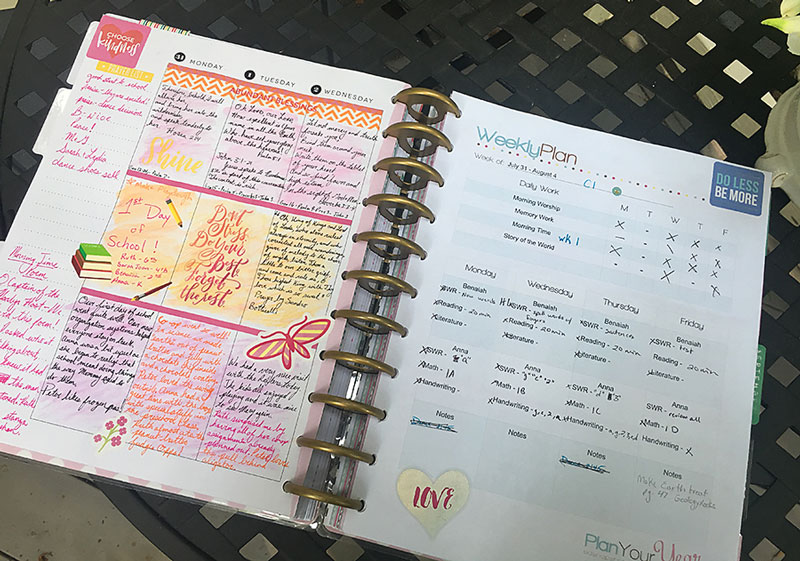A detailed description of the image would be:

An open weekly planner, secured with thick golden spiral rings, lies on a black, grated table outside on a porch. The planner displays meticulously filled-out sections for each weekday, Monday through Friday, with notably neat handwriting alternating in black, pink, and pinkish-red ink. On the left page, one can observe detailed plans for Monday, Tuesday, and Wednesday, complete with text, an image of a butterfly, and books, alongside notes on important events. The days of the week are further delineated with various markings: an 'X' on Monday and Wednesday, a dash on Tuesday and Thursday, and another 'X' on Friday. The header of the left page includes an inspirational quote: "Choose Kindness."

The right page is headed with "Weekly Plan" and features another motivational phrase, “Do less, be more,” ensconced in a blue, rounded square box. At the bottom right, a yellow heart encompasses the word "love" written in red. The rest of the space is filled with scribbled notes and some obscured names, signaling a very active and personalized usage.